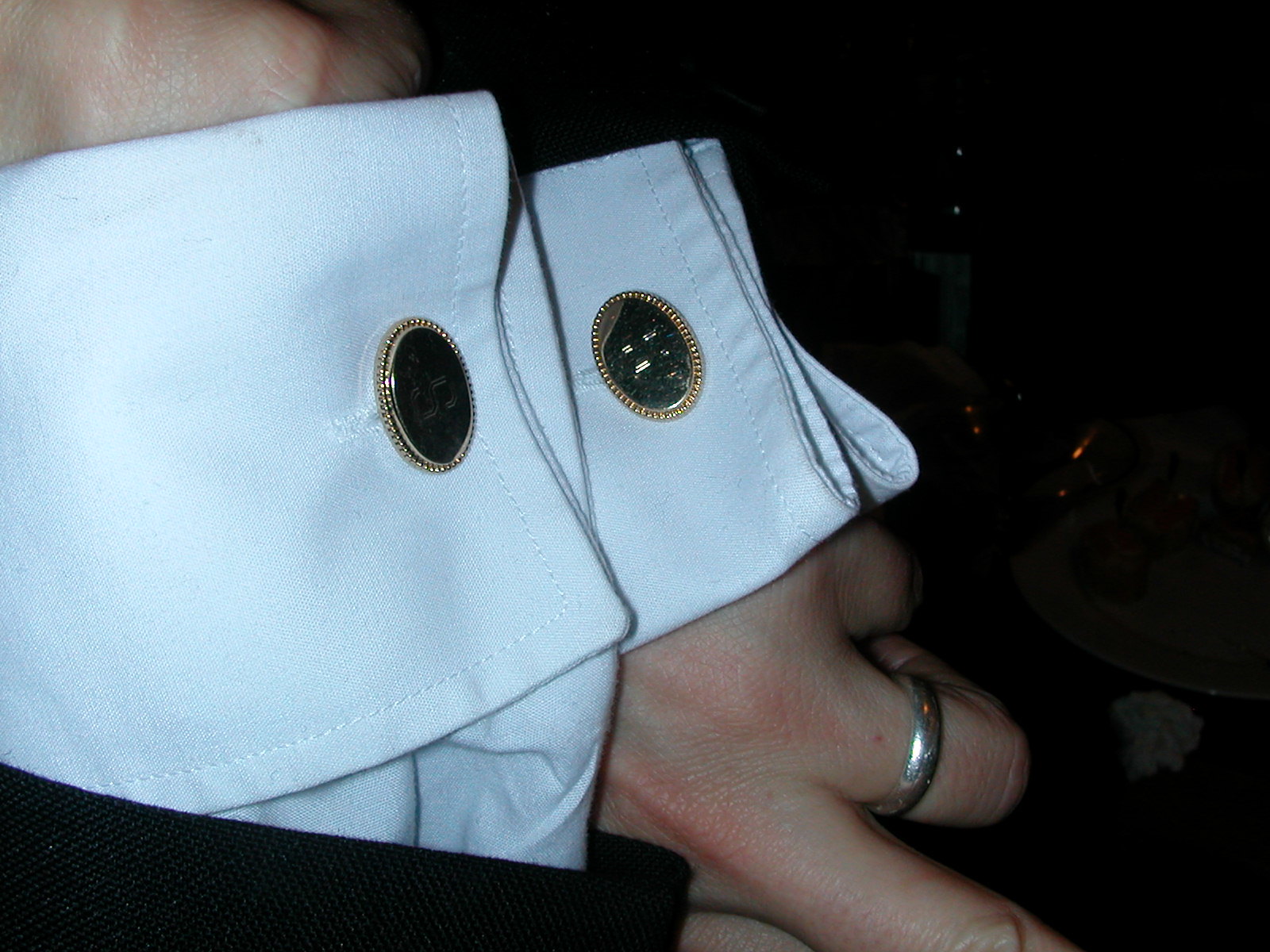The landscape-format, close-up color photograph captures an elegant, detailed view of a person's wrists adorned with high-quality fashion accessories. The focus is on the two meticulously designed gold cufflinks that embellish the crisp, white cuffs of a finely tailored dress shirt. The cufflinks command attention with their distinct oval shape, crimped border, and intricate dotted pattern, appearing almost cameo-like with an elusive engraved detail on their flat surface.

The photo reveals only a small fraction of the subject's hands, making it challenging to determine their gender, although one hand, presumed to be the left, displays a silver wedding ring. The person's hands are positioned somewhat unusually, with the left forearm pointing upwards and the right hand descending, bringing both cuffs and cufflinks into clear view. The immaculate white cuffs contrast sharply against the dark suit jacket visible at the sleeve ends, reinforcing the high-quality attire.

In the background, the image subtly hints at a dining scene, with a plate, a balled-up napkin, and a bottle partially visible against a dark backdrop. This sophisticated close-up not only highlights the elegance of the gold cufflinks but also provides a glimpse into the lifestyle and meticulous attention to detail of the individual wearing them.